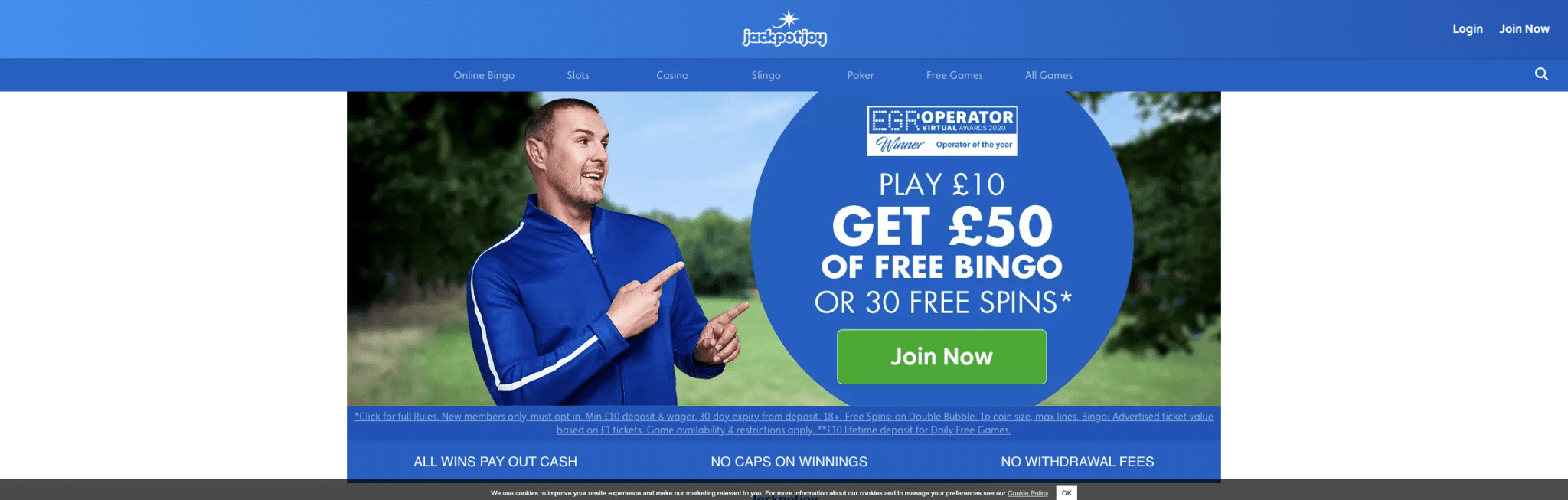The image appears to be a compressed screenshot of a company's website. The website features a prominent blue bar at the top with the company's logo centered, though the logo is too small to read. Below this, there's a darker blue navigation bar with seven indistinguishable options.

In the main section, there is a photo of a man standing outdoors in a field. He is wearing a blue Adidas-style sweater reminiscent of the 90s, with a single white stripe running up to the shoulder and a collar. The sweater is zipped up to the base of his throat, revealing a glimpse of a white undershirt beneath.

The man is pointing towards a circular, photoshopped advertisement that reads "EGR operator." Below this, the ad appears to offer a promotion: "Play €10, Get $50 of free bingo or 30 free spins." There is also a prominent green "Join Now" button beneath the text.